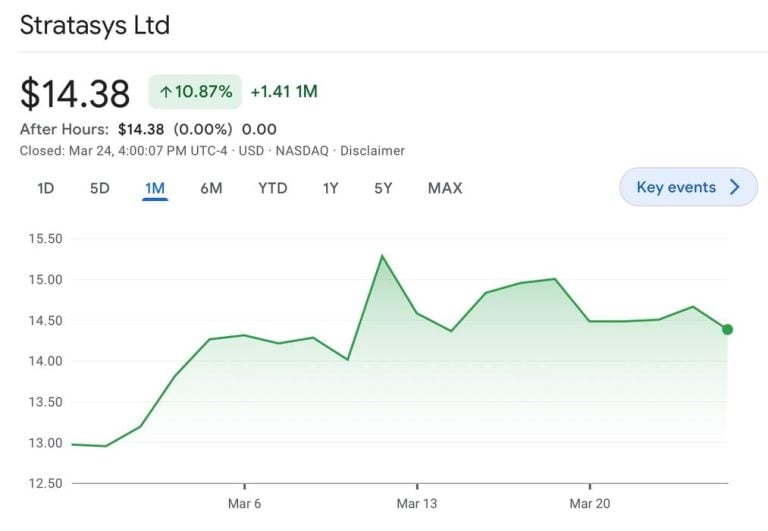The image features a screenshot of financial data for Stratasys Ltd (STRATASYS LTD), showcased against a white background. Highlighted prominently in the visualization, the stock price is displayed as $14.38, within a green rectangle indicating a 10.87% rise, denoted by an upward arrow. An additional light green rectangle shows a +1.41 increase for the month. As noted in the "After Hours" section, the price remains $14.38, with a negligible 0.00% change, recorded as of March 24 at 4:07 PM UTC-4.

Below the price data, a blue oval encloses the label "Key Events," next to which a right arrow points towards a timeline represented by clickable periods: 1D, 5D, 1M (highlighted in blue), 6M, YTD, 1Y, 5Y, and MAX.

A chart at the bottom of the image chronicles stock movements, marked with three key dates on the x-axis: March 6, March 13, and March 20. The y-axis tracks the stock price in increments of $0.50, ranging from $12.50 to $15.50. The chart shows a stock valuation of approximately $14.25 on March 6, rising to around $15.25 by March 13. Additional NASDAQ conventions and a disclaimer are visible, in keeping with financial reporting standards.